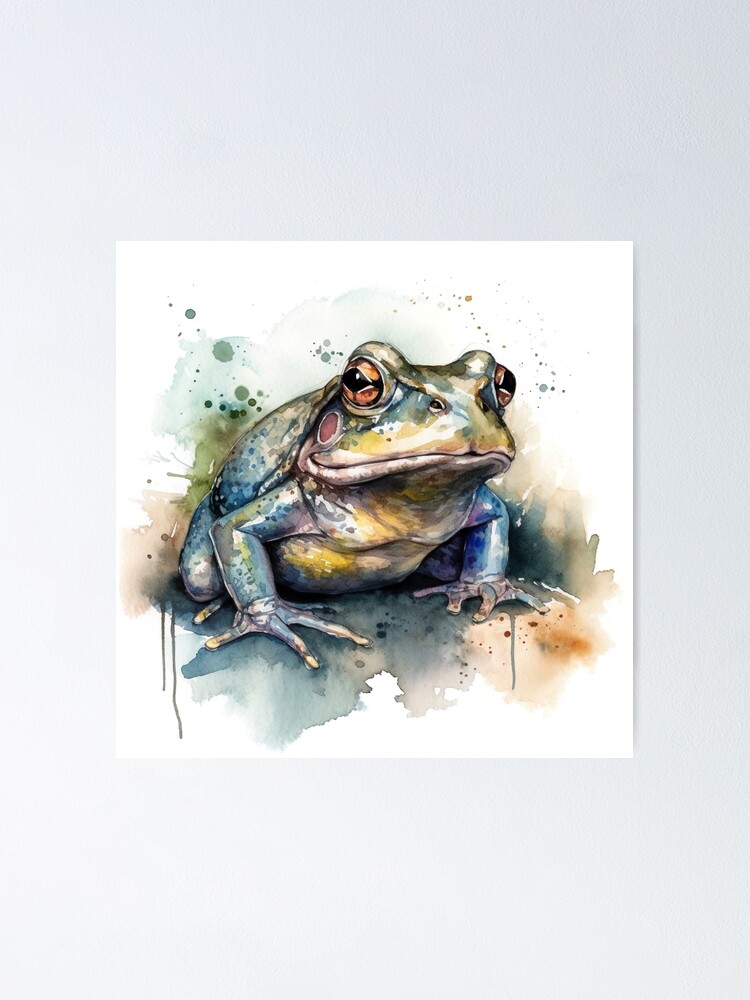The image is a detailed watercolor painting of a vividly colored frog, possibly a poison frog, depicted with a robust and hefty appearance. The frog stands prominently against a white square canvas, which itself rests on a light blue, textured background, perhaps a wall. Its body is a mosaic of greens, blues, yellows, and reds, with blue and purplish hues particularly noticeable on its arms and fingers that are spread out wide. The frog's large bulging eyes are directed towards the viewer, and it features a distinct red dot on its cheeks, reminiscent of rosy cheeks. Its back legs are primed for a leap, adding a sense of dynamic motion to the artwork. Surrounding the frog are splotches and spatters of various colors—blue, green, red, and others—contributing to a vibrant and lively composition. There are also paint drips and splatters, enhancing the whimsical and dynamic feel of the painting.